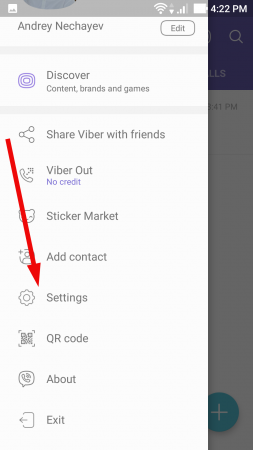A smartphone screenshot taken at 4:22 PM displays several key interface elements. The status bar at the top indicates a nearly full battery, three out of four bars of cellular signal strength, and a full Wi-Fi signal. A prominent popup window in the center presents options such as "Entry," "Net Show," and "Net Retrieve," with an "Edit" button beside it. Below the popup, a heading reads "Discover Content, Brand, and Games."

Further down, there's a white box featuring a share icon with the text "Share Viber with Friends." Beneath this, a phone icon labeled "Viber Out, No Credit" appears, followed by a section for the "Sticker Market." The next option, "Add Contact," precedes a gear icon leading to "Settings," which a large red arrow prominently points toward. Additional options below include "QR Code" with its corresponding icon, "About," and at the very bottom, "Exit."